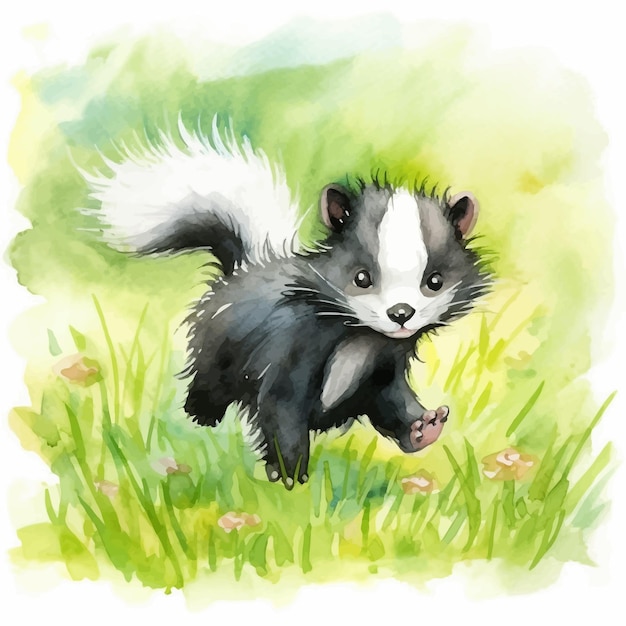This is an enchanting watercolor painting of an adorable baby skunk. The skunk, depicted with a characteristic black body and a prominent white stripe running from its head to its fluffy tail, is clearly identified as a baby by its smaller, rounder, and fluffier appearance. Its endearing features include a white patch on its chest, a white line between its eyes, and around its nose and mouth, with cute little whiskers that give the impression of a gentle smile. The painting beautifully captures the skunk's pink little pads and toes, as well as the loose, fluffy hairs around its tail and body. The background, rendered in blurry green hues with hints of blues and yellows, suggests a grassy area accented by pale, brownish-yellow blossoms. Though lacking in detail, the background effectively directs the viewer’s attention to the skunk, the focal point of this charming and lovely piece of art.